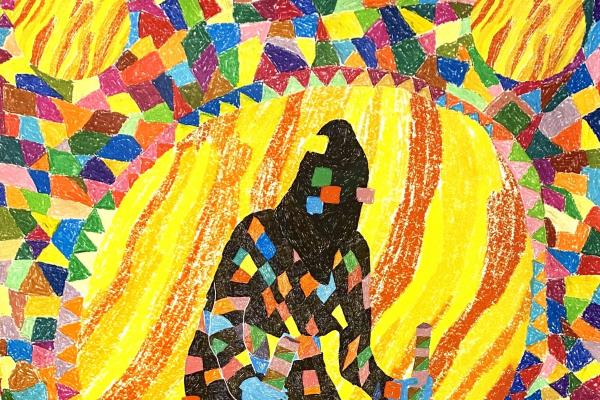The artwork portrays a highly abstract scene, likely crafted with crayons, featuring vivid and varied colors. At the core is a hooded figure centered at the bottom, depicted in black with geometric patterns of small colored rectangles, squares, and triangles in shades such as yellow, green, red, blue, pink, and orange. The figure's belt is composed of reverse triangles arranged vertically, adding to its intricate design. Encircling the figure is a yellow ring with wavy orange lines extending outward, bordered by additional triangles. The backdrop transitions into a more chaotic composition with clusters of triangles and rectangles in an array of colors like pink, purple, brown, and green. Two yellow circles occupy the top left and right corners, imitating suns, enhancing the abstract and vibrant nature of the piece.